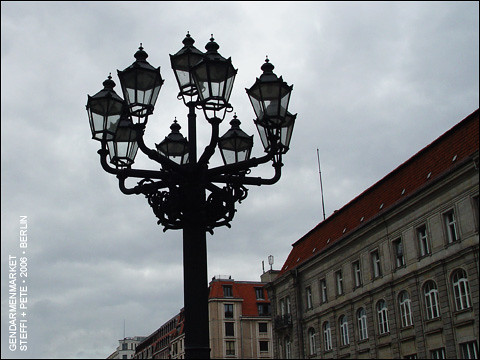This detailed color photograph captures a striking, medieval-style lamppost located in Berlin, Germany, silhouetted against a cloudy, gray sky. The lamppost, painted a sleek black, features a complex design with nine lanterns. Each lantern is adorned with clear glass sides, topped by black lids with ornate scrolls or spears. The central pole, which holds four cross arms, extends variously placed lanterns, adding to the intricate appearance of the structure. In the background, partially seen to the right, is a grand Victorian-style building with sandy-colored brickwork and a dark clay roof, adding to the historical ambiance of the scene. Text visible in the bottom left corner of the image reads "Den Darmen Market Steffi + Pete 2006 Berlin," confirming the location as a vibrant market street in Berlin.